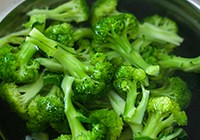This detailed photograph features a vibrant green array of steamed broccoli florets, carefully arranged within a bowl that appears to be black or dark-colored. The photo, though small, captures the intricacies of the broccoli well, with the florets displaying a vivid contrast between the darker green tops and the paler green stalks. The broccoli is piled high and scattered in a random, yet natural pattern, filling the bowl and overlapping into one another. The surface of the broccoli has a slightly moist appearance, suggesting it has been freshly cooked. The light reflecting off the florets highlights parts of the texture, adding depth to the composition. The edges of the bowl can be seen, and there are lighter areas in the top left and right corners of the image, indicating the bowl’s depth. Overall, the photograph captures a rich, detailed, and inviting view of the broccoli, emphasizing its freshness and vibrant color.